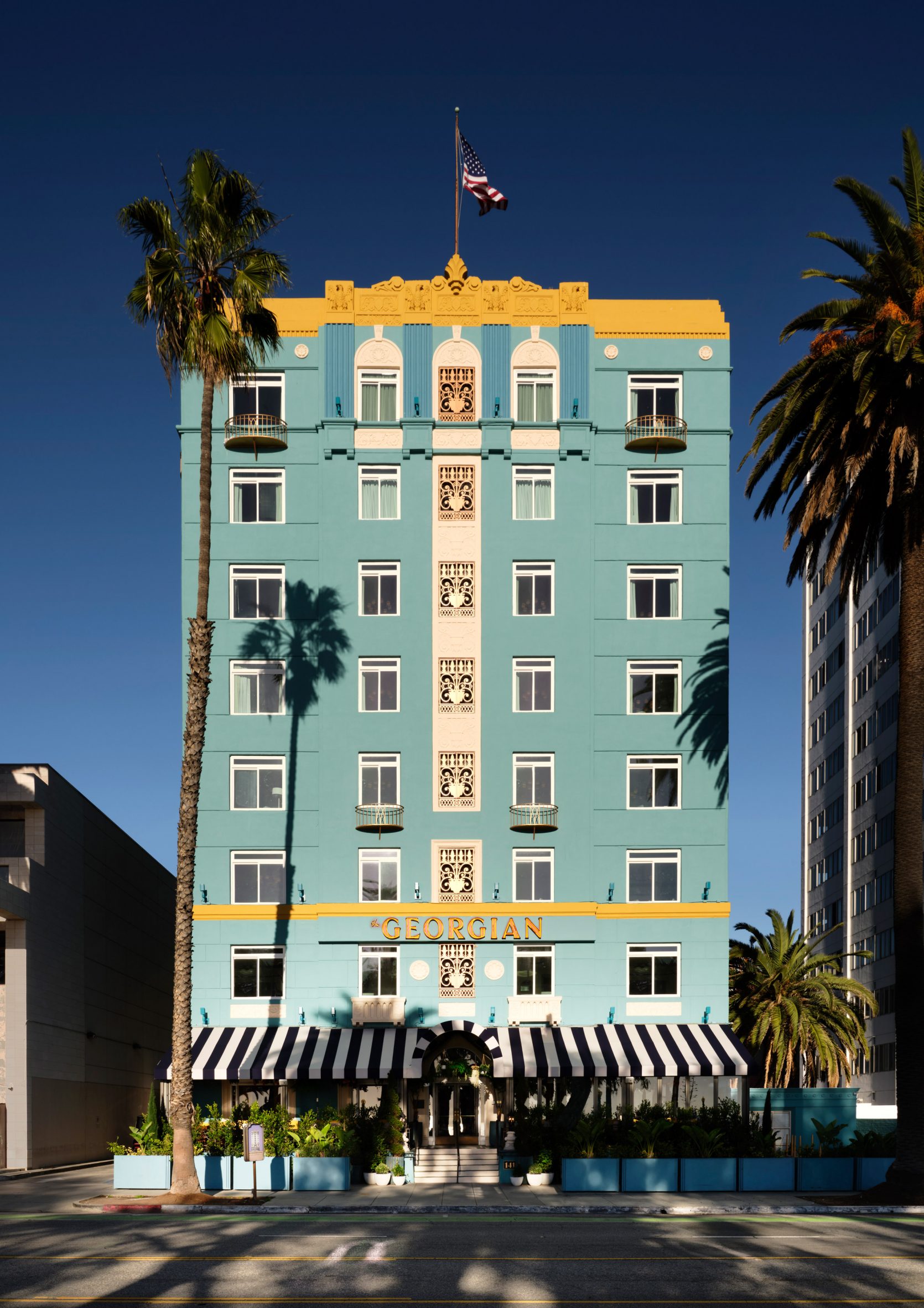This is a photo of a tall building, specifically eight stories high, likely a hotel, characterized by its distinct architectural details and color scheme. The building is primarily painted a teal blue or turquoise color, with a striking mustard-yellow section at the top adorned with ornate details. An American flag prominently tops the structure, waving from the center of the roof. The facade features neatly aligned windows in horizontal rows—four per each of the eight stories. Interspersed in the middle of the blue facade is a vertical beige stripe with intricate wrought iron detailing.

The first floor boasts a black and white vertically striped awning above double front doors, adding to its classic appeal. Above this entrance, in gold letters, reads "Georgian," marking the establishment's name. Surrounding the base of the building, particularly on the second story, are blue planters brimming with various greenery, enhancing the frontage with natural elements. To the left of the building stands a prominent, tall, and skinny palm tree, casting its shadow on the facade, while more palm trees can be seen off to the side, complementing the hotel's surroundings. The sky above transitions from a darker to a lighter blue, which serves as a picturesque backdrop to the building. The entire scene is bordered by gray asphalt with yellow road lines, setting the structure within an urban landscape. The building is flanked by a shorter structure on the left and another of similar or greater height on the right.